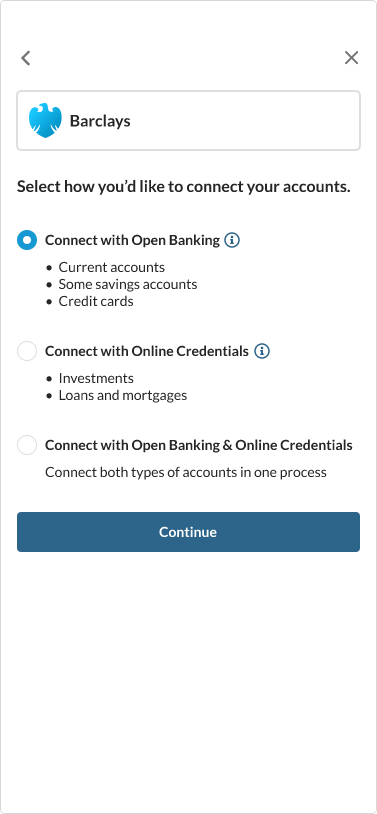The image is a vertically oriented rectangular graphic with a white background. Near the top-left corner, slightly offset from the edge, is a small left arrow symbol, resembling a less-than sign. In the top-right corner, an "X" symbol is present.

Below this, a horizontal rectangular section is outlined with a light gray border. Inside this section, the word "Barclays" is prominently displayed in black bold font. Situated to the left of the word "Barclays" is a turquoise logo that appears to depict a bird, although the exact design is unclear.

Beneath the Barclays logo and text, another line of black bold text reads: "Select how you'd like to connect with your accounts."

Following this instruction, there is a small white circle with a thicker, turquoise outline. To the right of this symbol, bold black text reads: "Connect with Open Banking." Adjacent to this text, an information icon represented by a white letter "i" in a blue circle is displayed.

Below this option, a list indicated by black bullet points enumerates: "current accounts," "some savings accounts," and "credit cards."

Next, another connection option is presented with an empty circle, followed by bold black text stating: "Connect with online credentials." A turquoise information icon, represented by a "i" in a turquoise circle with a white background, is placed next to this text.

The associated list of account types for this option, marked by black bullet points, includes: "investments," "loans," and "mortgages."

A third connection choice follows, signified by an unfilled circle and bold black text that says: "Connect with Open Banking and online credentials." Below this, explanatory text in regular black font reads: "Connect both types of accounts in one process."

At the bottom of the section, a horizontal rectangular teal button stretches across, with the word "Continue" in white font centered within it.

The remainder of the image consists of a blank white space, all enclosed within the light gray border.